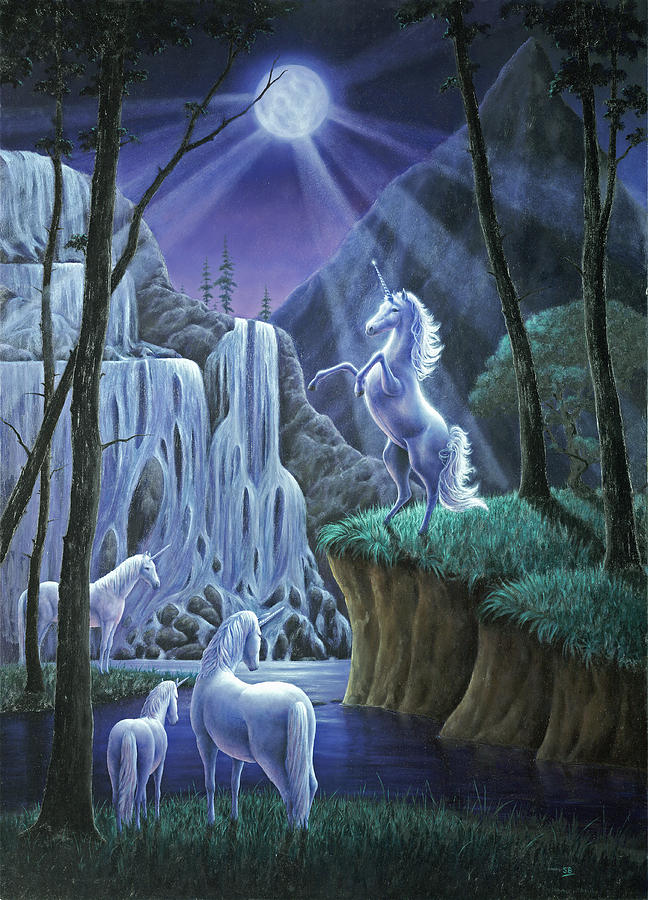This is a detailed color illustration in a fantasy style, depicting a tranquil, moonlit night scene. The full moon is positioned at the top center, casting visible rays that illuminate the landscape below. Dominating the scene on the left is a grand, tiered waterfall cascading over rocks into a large body of water. Emerald green grass carpets the foreground and lower hillside, surrounded by sparse, tall trees whose tops are cropped from the image. 

In the foreground, a white unicorn is majestically rearing up on its hind legs atop a grassy hill. Nearby, another larger unicorn stands, gazing down at the water, while a smaller foal stands to its left. A third unicorn is positioned to the middle left, appearing to watch the rearing unicorn. The scene is bathed in cool tones, creating a serene, enchanted atmosphere with the moonlight as the sole source of illumination.